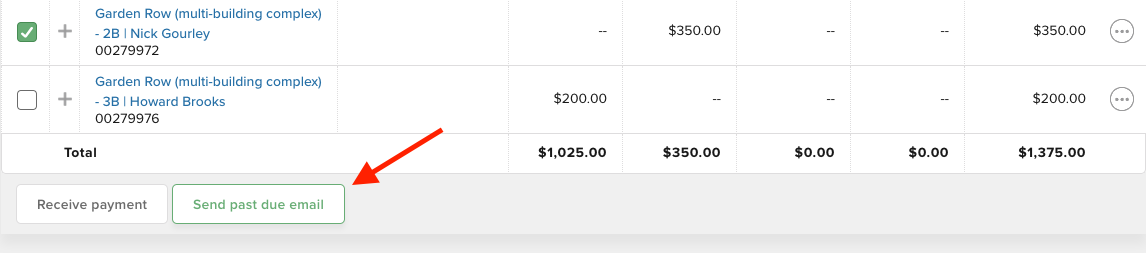The image depicts a detailed transaction record presented in a small rectangular box against a white background. On the far left of the box, there are two checkboxes, with the first one checked. Adjacent to each checkbox is a plus symbol. 

In the first row with a checked box:
- The text reads "Garden Row (Multi-Building Complex)".
- This is followed by the name "Nick Gourley" (spelled G-O-U-R-L-E-Y) and a transaction ID "00279972".
- Moving to the right, the five columns show specified values, with the second column displaying $350 and the fifth column also listing $350.

The second row:
- Also labeled "Garden Row (Multi-Building Complex)", this entry specifies "3B Howard Brooks" with a transaction ID "00279976".
- The first column lists $200, and similarly, the fifth column lists $200.

Below these rows, under the "Garden Row" section, the term "Total" is distinctly highlighted:
- The totals are 1025 for the first column, 350 for the second column, zero for the third and fourth columns, and 1375 for the fifth column. These totals are emboldened in black for emphasis.

Lastly, a red arrow points to a separate box that contains the text "Send Past Due Email" written in green.